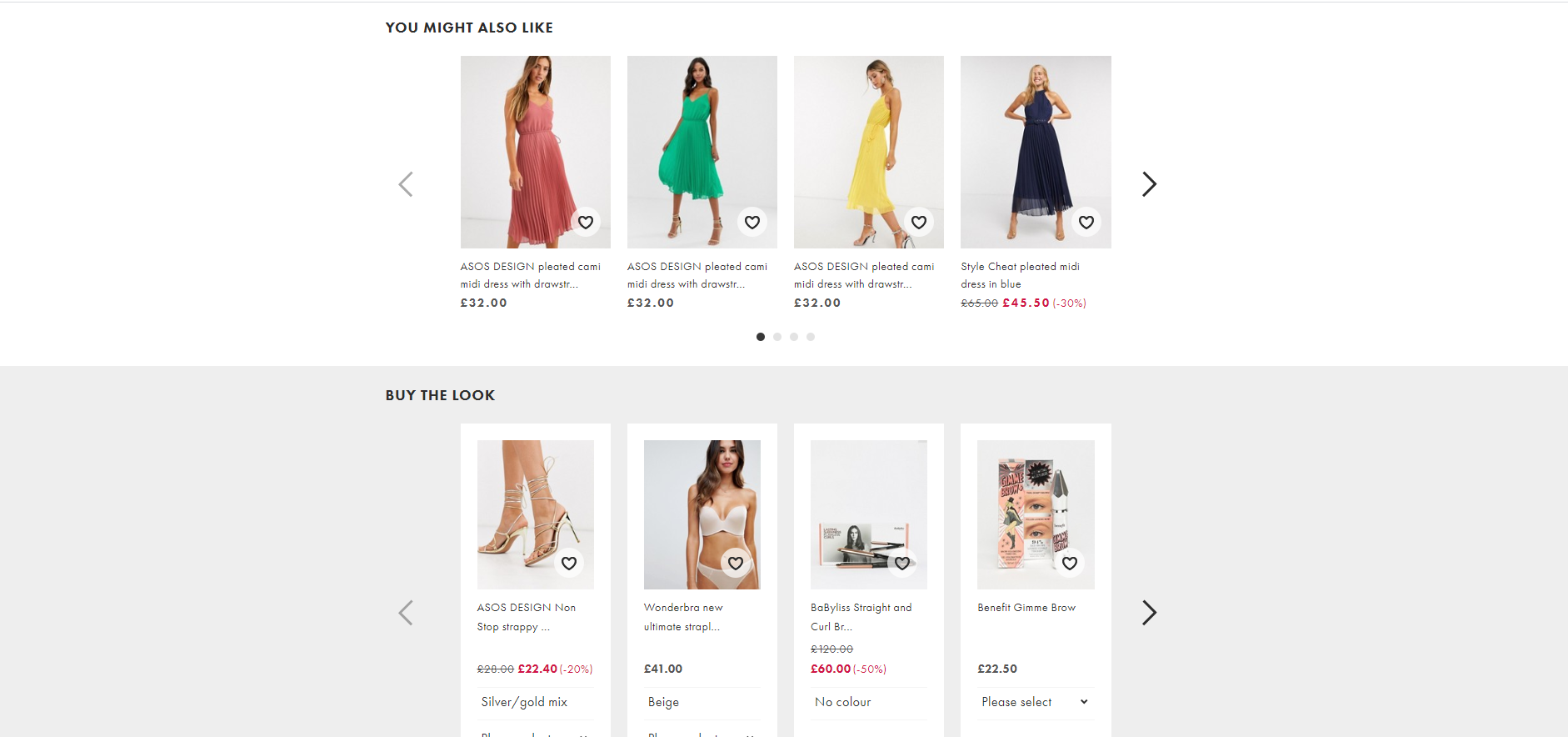This is an image of a cropped screenshot from a clothing website showcasing a selection of dresses and complementary products. The top half of the image features a white background with four centrally-aligned dress thumbnails. Below each dress thumbnail, the designer's name, the dress name, and its price are displayed. Each thumbnail also has a heart icon and a circle on the bottom right for favoriting the dress. Arrows are present on the left and the right sides of the thumbnails, allowing users to scroll through the dress options like in a carousel.

The bottom half of the image has a gray background and prompts viewers with "Buy the Look" on the top left. This section similarly displays four product thumbnails, which include items like high heels, shoes, undergarments, and makeup. The format mirrors the dress section: a heart icon for favoriting is on the bottom right of each thumbnail, with the designer's name, the product name, and the price listed directly below the thumbnail. Additionally, these product thumbnails indicate the available colors of the items, with the last product featuring a dropdown box that says "Please select."